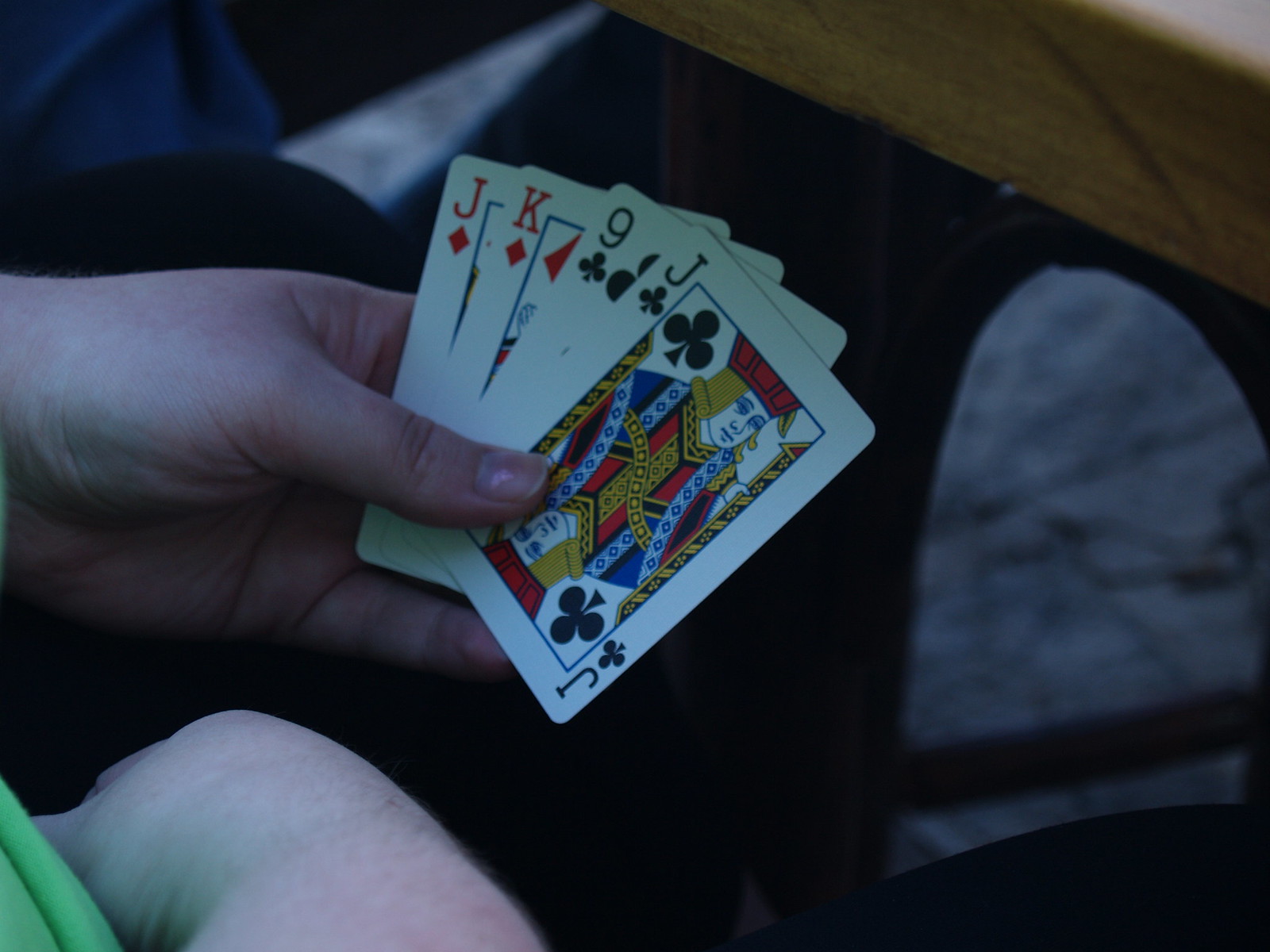In this detailed and clear image, a person dressed in a green shirt is holding four playing cards in their left hand. These cards are, from left to right: the Jack of Diamonds, the King of Diamonds, the Nine of Clubs, and the Jack of Clubs. The person’s left thumb is horizontally placed across the four cards, with the hand noticeably cupped as it grasps the rest of the deck. The individual’s right arm is wrapped around their belly. This detailed capture also reveals a patch of hair on the person’s right forearm, as well as creases in their skin, suggesting the clarity of the photo.

The scene is set over a table that has an object with a bent-up corner, possibly a piece of paper or a card. The texture and slight lift of this corner are clearly visible. Among the elements on the table is a gray, oval-shaped image with a black band running across it, whose purpose or design remains unclear. This gray element and the bent-up piece both share a similar color. Additionally, part of another garment, possibly a blue T-shirt, is visible in the scene.

An intriguing detail adding to the context is the hint of pink nail polish on the left thumb nail, suggesting the hand might belong to a woman. The high-definition nature of the photograph not only captures the vibrancy of the colors but also the finer details such as the individual hairs and skin creases, making it a remarkably vivid image.